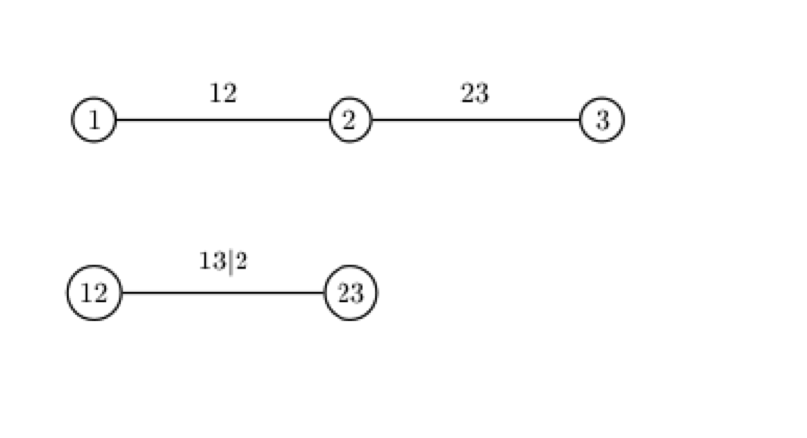The image depicts a scale or diagram featuring a series of numbers and lines. There are two primary horizontal lines: the top line and the bottom line. On the top line, there are three sections, each marked by black circles containing the numbers 1, 2, and 3. These circles are connected by straight lines. Specifically, the circle with the number 1 is located at the far left-hand side, linked to the circle with the number 2 by a line. This line bears the number 12 above it. Similarly, the circle with the number 2 connects to the circle with the number 3 by another line, with the number 23 above it.

Below this, the bottom line mirrors the top line's layout with black circles containing the numbers 12 and 23. This line is equidistant from the top line and also has the number 23 above it. Above this bottom line, there is text that reads "13-2" in a slightly faded font, suggesting the printer may have been running low on ink. The text and lines are all black, and there is no other content or background in the image. The overall visual is simple and clear, focusing solely on the numbers and their connections.